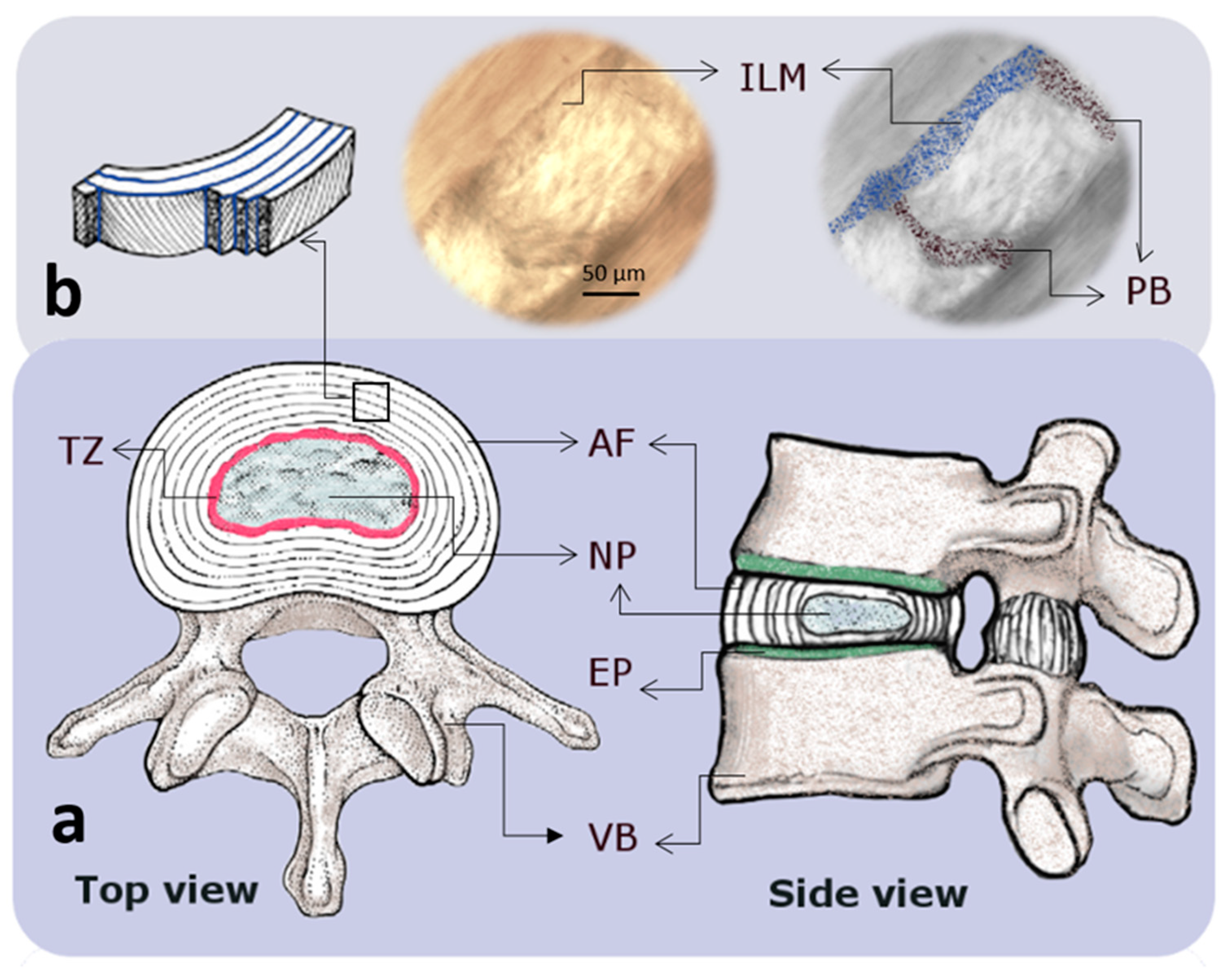This detailed infographic, in landscape orientation, depicts a labeled diagram of various views of a spinal disc or bone section with accompanying notations. The top portion features a light purple background with a labeled section "B" on the top left corner, illustrating a black and white cross-section of a circular bone or spinal disc. Adjacent to this is a detailed, round color illustration of the bone, predominantly tan with blue and black markings. It is annotated with text such as "50 UM" and "ILM," and includes arrows labeled "PB" pointing to various sections. Below the main illustrations, the infographic transitions to a darker purple background, showcasing two views of a spinal structure. On the bottom left, a "top view" is labeled "A," depicting the bone with internal structures denoted by abbreviations like "TC," "AF," "NP," "EP," and "VB," with detailed lines in blue. The bottom right presents a "side view" of the same structure, also with notations and arrows, providing a comprehensive look at the internal layers and composition. The style is a detailed, color illustration combined with text annotations, highlighting different angles and layers of the spinal bone.